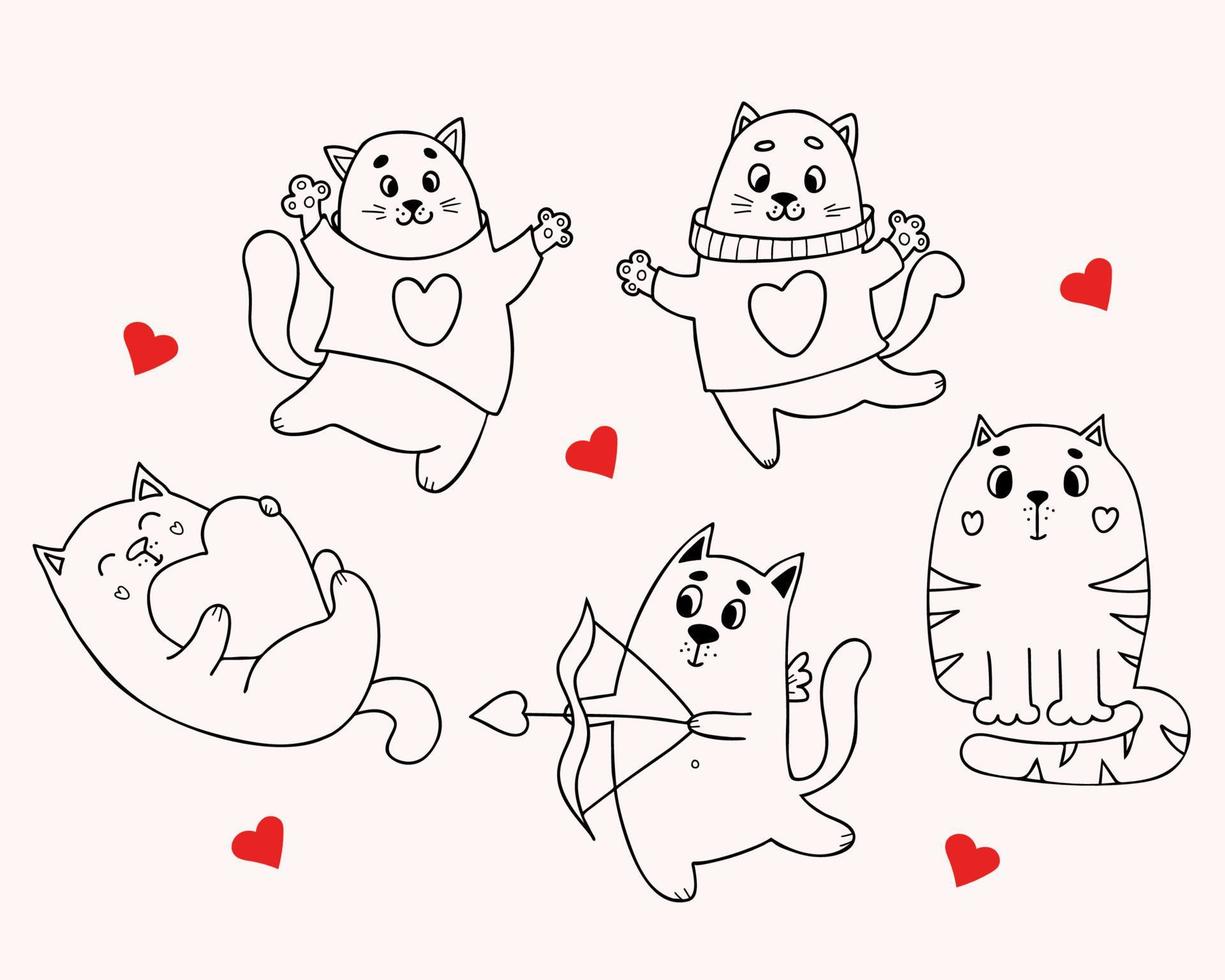This is an illustration of five cartoon cats on a very light pink background, accentuated by small red hearts scattered around them. Drawn in black and white, these whimsical felines are depicted in various playful poses. The two cats at the top have pointy, cat-like ears and three-toed paws extending from sweaters adorned with heart motifs, complete with tails peeking out. Below them, the scene features three more cats. One on the left is lying down with its eyes closed, cradling a heart-shaped pillow. The middle cat, armed with a bow, is aiming a heart-shaped arrow. The third cat, distinctive with stripes and small hearts on its cheeks, sits serenely with its tail curled in front. The illustration combines a blend of cuteness and charm, enhanced by the presence of five heart symbols.